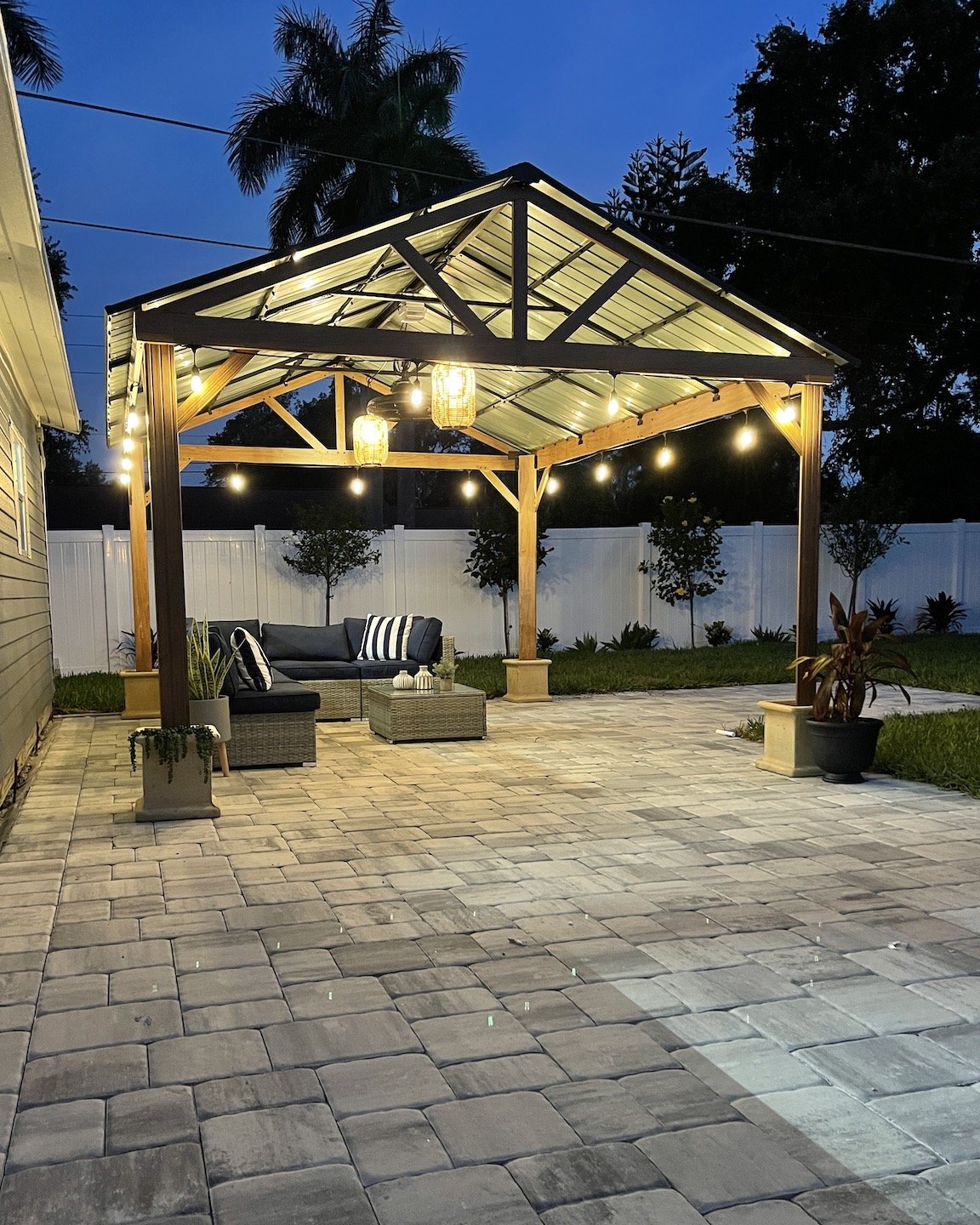The image captures a serene backyard scene taken at night just after sunset, with the sky painted in a dark blue hue. The central feature is an inviting outdoor covered area with a triangular roof made of plain metal. The structure is supported by sturdy wooden beams, forming a simple yet elegant frame. Hanging from the rafters are delicate outdoor lights and chandeliers that softly illuminate the space below.

Beneath the cover, there's a cozy L-shaped wicker sectional with navy blue cushions, complemented by white stripes on the back cushions. A matching gray wicker coffee table adds to the cohesive design of the seating arrangement. The ground beneath this setup is paved with irregularly shaped stones in varying shades of light to dark gray.

The backyard is bordered by a white plastic fence that separates it from adjacent properties. The fence is lined with small trees and bushes, with tall palm trees and telephone poles rising above it, silhouetted against the dusky sky. On the left side of the image, part of the residence is visible, featuring gray panel siding and illuminated windows. The entire scene exudes a tranquil, welcoming atmosphere, perfect for evening relaxation.